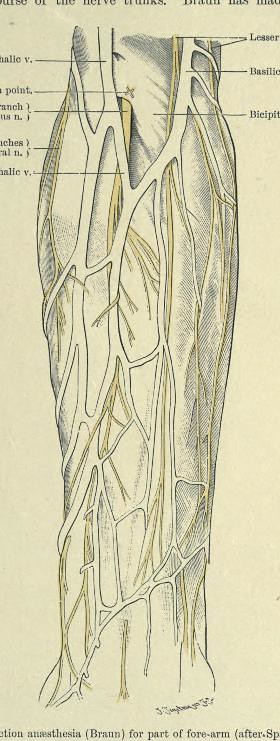This detailed anatomical drawing appears to depict a forearm, showcasing veins, arteries, and musculature. The illustration adopts a "see-through" style, revealing the various internal structures. The veins are rendered in white, while the arteries are highlighted in yellow, set against gray-toned musculature. The background resembles light yellow archival paper. At the top, the drawing features two labeled columns; the left includes terms like "PHLICV" (possibly a vein), "point," "branch," "N S N.", "inches", "ALN.", and "ALICV.", likely referring to veins. The right column includes labels such as "lesser," "basilic," and "bicipit." The bottom of the image displays partially obscured text: "E-T-I-O-N anesthesia B-R-A-U-N for part of forearm (S-P)." The entire illustration seems to be executed in pencil or charcoal, aimed at providing an educational view of the forearm's internal anatomy.